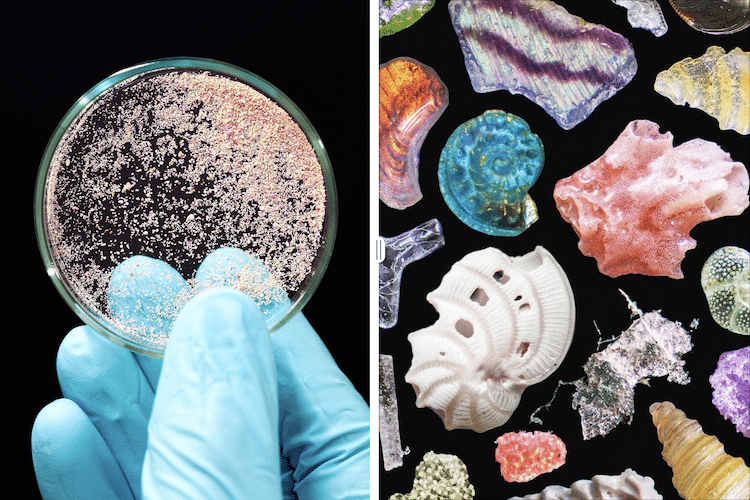This composite photograph features two images set against a black background. On the left, a blue latex-gloved hand, appearing to be a right hand, holds up a Petri dish. The dish, rimmed with gray, contains what seems to be small pink particles—possibly sand or salt—clustering predominantly on one side. To the right of this image, an assortment of various shells and coral pieces is meticulously arranged. These marine specimens exhibit a vibrant array of shapes, colors, and sizes: a blue conch shell, peach-colored coral fragments, horn-shaped and transparent glass-like shells, as well as snail and oyster shells. Notably, there are also unique pieces like a yellow conic shell with horizontal stripes and a slightly lavender shell fragment with big purple stripes at the top, creating a visually captivating contrast against the solid black backdrop.